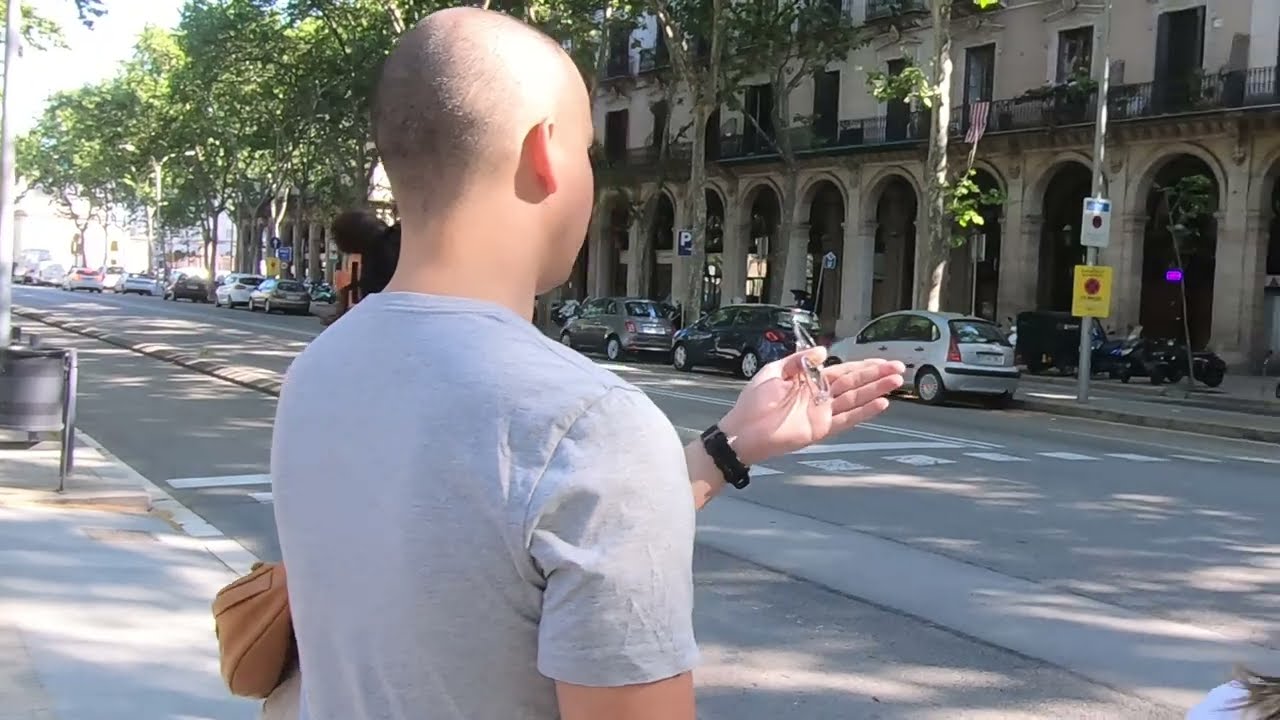In the photograph, a man sits prominently in the foreground on a city sidewalk. Positioned slightly left of center, he faces away from the camera, wearing a light gray, short-sleeved t-shirt. His head, appearing mostly bald with some fine hair, catches sunlight on its top right. The man stretches out his left hand as if gesturing towards something across the street. He sports a black wristwatch and holds a pair of sunglasses hooked onto his thumb. To his left side, he carries a small, light brown backpack or handbag.

Partially obscured behind him, a woman with her hair in a bun is barely visible. A gray garbage can sits on the sidewalk to the far left of the image. The city street ahead is lined with parked cars, including a white car, a dark blue car, and a silver car, while no vehicles pass in front of him at the moment. The street stretches towards cream-colored buildings adorned with arches on the ground floor and black railings on the second. The sun peeks out from the top left, casting a mix of light and shadow across the scene. Additionally, an array of trees lines the sidewalk, their foliage contributing to the dappled sunlight patterns that fall across the pavement. On the left-hand side of the background, a tall pole with traffic instructions can be seen, featuring both yellow and white signage.